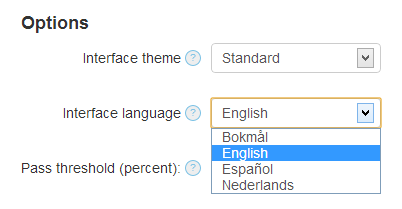This screenshot captures a concise interface options page, likely from a settings menu on a website or application. The available options seem limited, focusing primarily on interface customization and language preferences.

The visible settings include:

1. **Interface Theme**: The selected option here is "Standard," suggesting it might be a default or common theme without additional details provided in this view.
2. **Interface Language**: This section presents a dropdown menu for language selection, with the current selection highlighted in blue. The available language choices include:
   - **Bach Mai**
   - **English** (currently selected)
   - **Español**
   - **Nederlands**

3. **Pass Threshold (%)**: This setting is somewhat obscured by the language dropdown menu, preventing a clear view of its selectable options. The term refers to a percentage-based threshold, though its specific function remains unclear from this screenshot alone.

The overall simplicity of the options indicates that this may be an interface designed for straightforward language and theme customization, enhancing usability for users who require basic personalization.